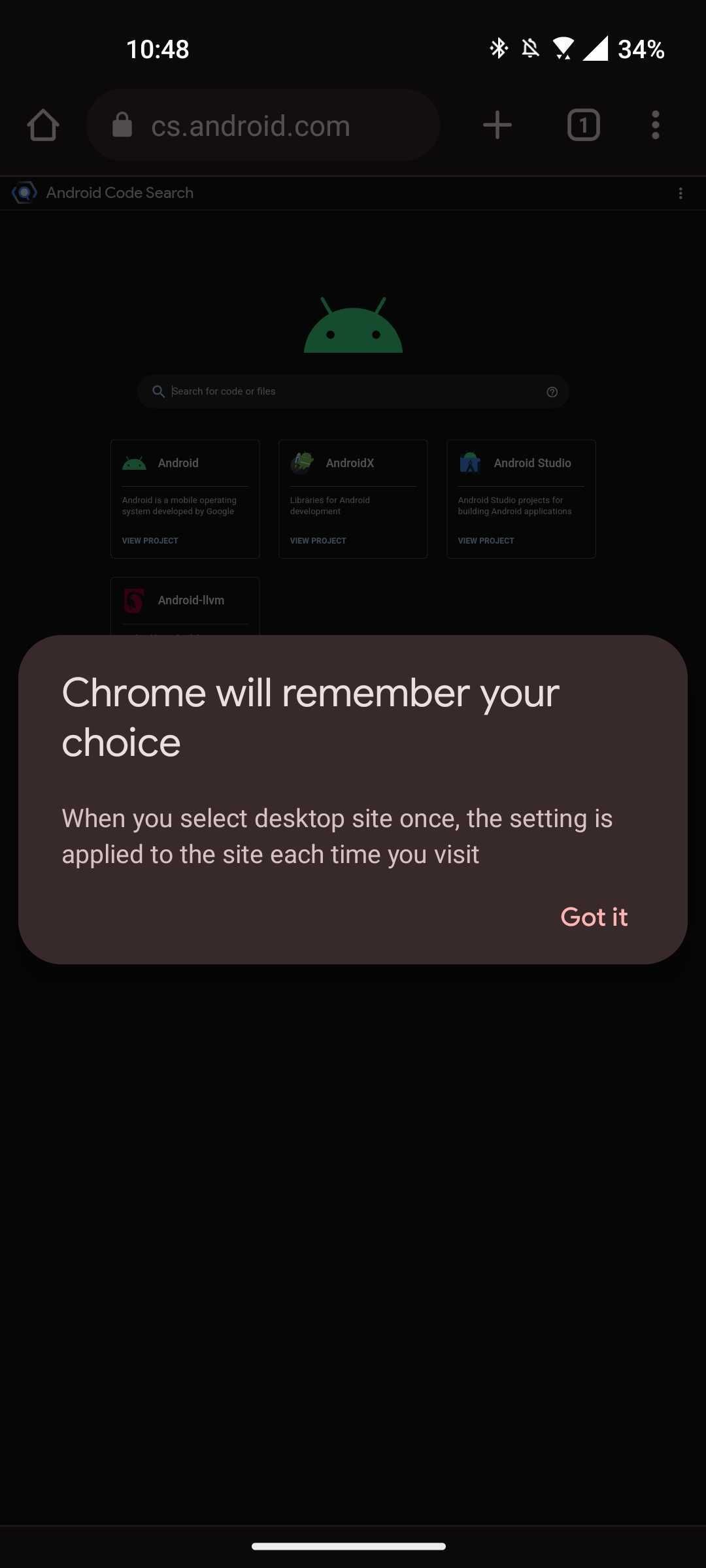The image is a screenshot from a smartphone displaying a pop-up message in the center. The message from Chrome informs the user that the browser will remember their choice to view sites in desktop mode once the setting is applied, ensuring this preference is retained for future visits. At the bottom right corner of the pop-up, there is a button labeled "Got It."

Behind the pop-up, the phone's browser is visible. The address bar at the top reads "cs.android.com," and the current time displayed in the upper right corner is 10:48. The battery percentage indicator shows the phone is at 34% charge.

Below the address bar, the page header reads "Android Code Search" accompanied by the Android alien logo. A search bar follows, with the placeholder text "Search for code or" featuring a slightly pixelated word beneath it. Further down, there are four categorized sections listed as "Android," "AndroidX," "Android Studio," and what appears to be a partially obscured or pixelated "Android MVM."